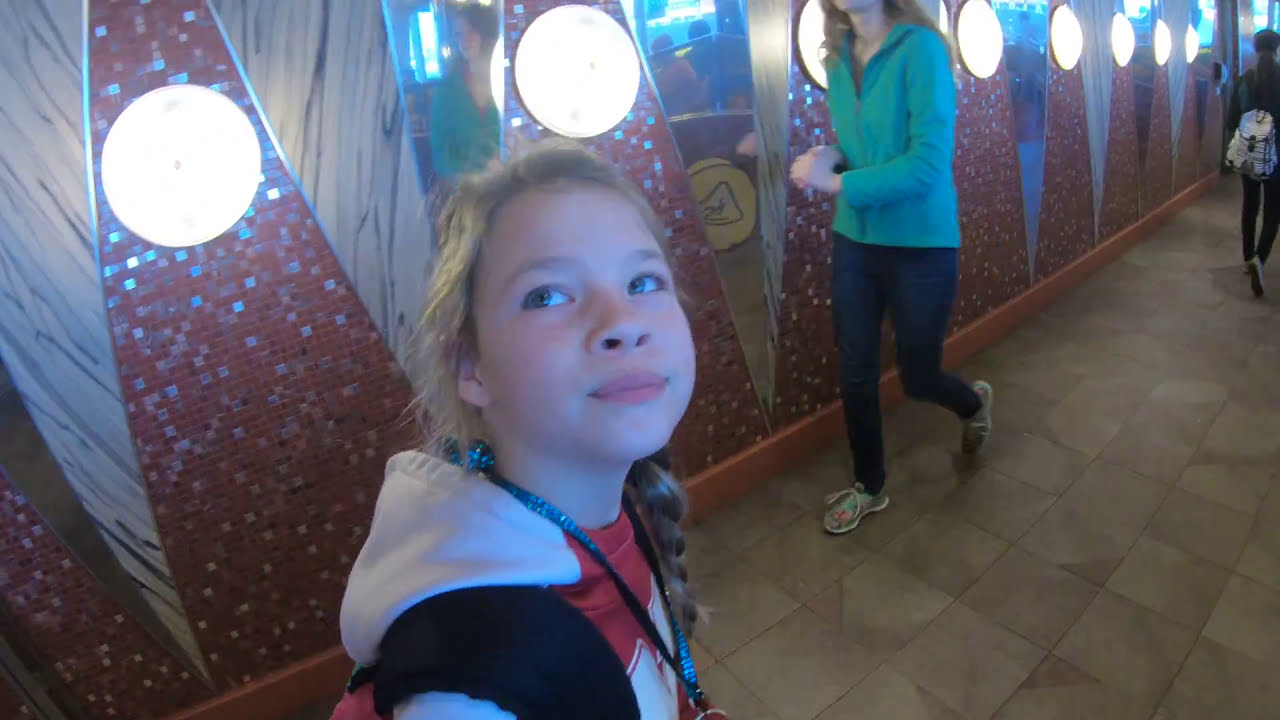The image captures an interior walkway filled with activity. At the center, slightly to the left, stands a young girl, likely between 5 to 7 years old. She has blonde, slightly messy hair pulled into an unbraided ponytail draped over her shoulder. The girl is intently gazing upwards towards the top left corner of the photograph with her blue eyes. She is dressed in a red and white hoodie layered over a red t-shirt. A red backpack with black straps is slung over her shoulders, and a blue metallic lanyard ending in a metal ring hangs around her neck.

The walkway beneath her and throughout the corridor is covered in gray tiles, leading to other individuals moving in various directions. Notably, a person dressed in blue jeans, a light blue jacket, and gray and blue tennis shoes walks opposite the girl. To the right side of the image, another individual clad in tight black pants, a black jacket, and a white backpack strides forward.

The background is a visually striking wall composed of red tiles interspersed with shimmering silver triangles. These reflective surfaces create the impression of a dancing mosaic, enhanced by circular white lights scattered across the wall. The scene hints at a lively, well-lit environment, likely a public indoor space such as a museum or a hotel lobby.